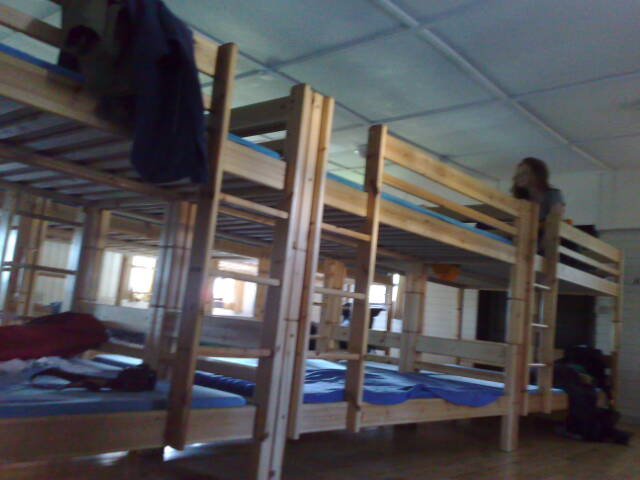The photograph depicts what appears to be a dormitory, hostel, or camp setting with multiple wooden bunk beds arranged in rows. The bunk beds are made of light brown wood and each unit includes a built-in wooden ladder. Blue sheets or blankets are visibly spread over the lower bunks, and on the bed closest to the camera, a red object is noticeable. Hanging from an upper bunk are some blue and green clothes, suggesting personal spaces. The lighting in the room is dim with a slight blue tint, and natural light filters in through the windows at the back. A woman with long hair, possibly red or appearing red due to the lighting, is seated on an upper bunk in the front row, beside a built-in ladder. She is looking out to the left. The ceiling is low and has a square grid pattern, similar to a drop ceiling, creating a somewhat compact and confined atmosphere. The presence of personal belongings on several of the bunks indicates that the beds are currently in use.